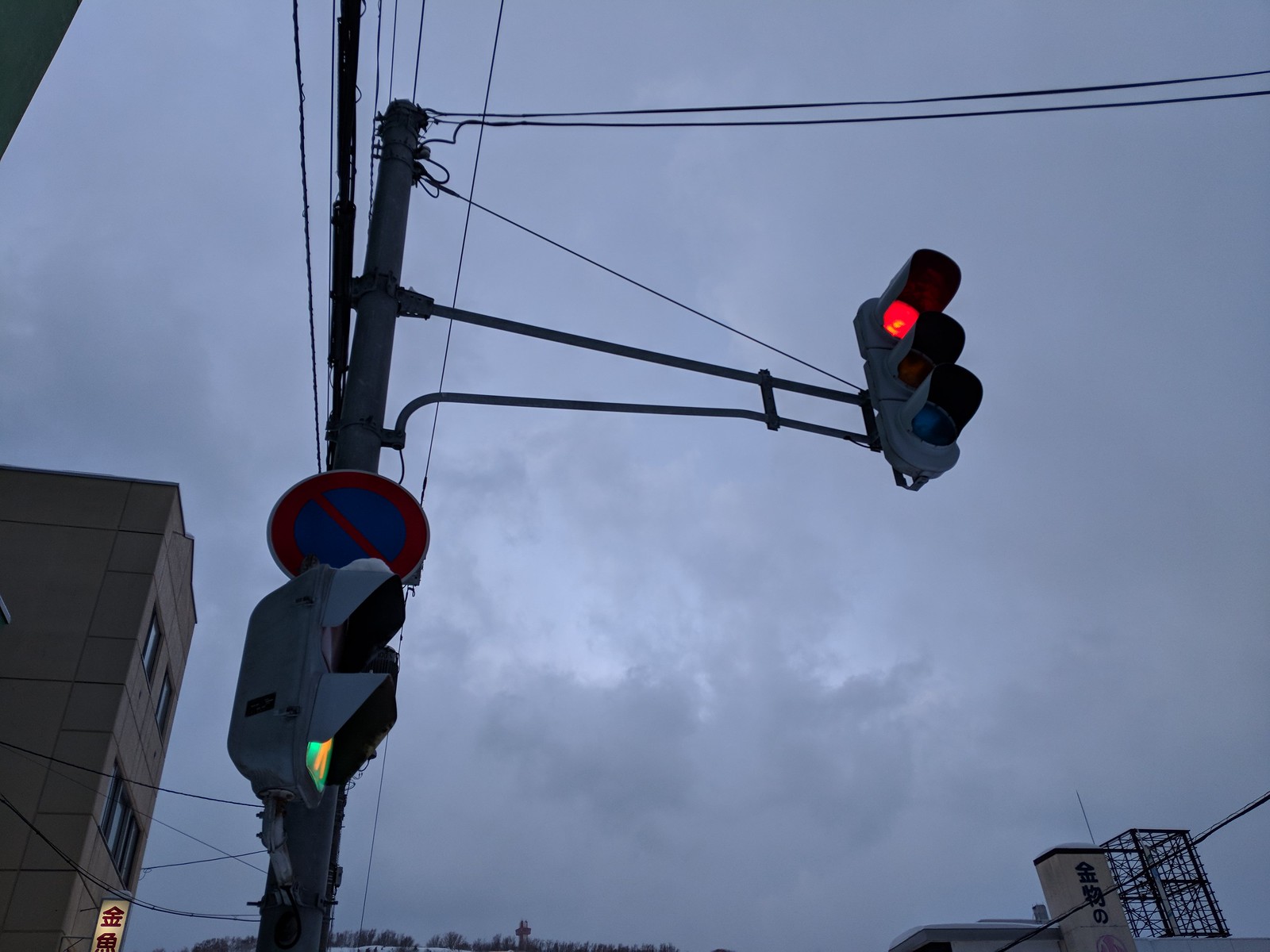The photograph, taken at dusk, captures a cloudy, darkening sky with an imminent storm-like atmosphere. The vantage point is looking upwards, focusing on a tall telephone pole situated on the left side of the image. Attached to the pole near the bottom is a blue-and-red circular sign. Extending from the pole, a thin arm holds a traffic light, with its red light illuminated at the top. Surrounding the traffic light are cylindrical black visors approximately two inches long. Atop the pole, electric wires stretch vertically and horizontally, contributing to a web-like appearance.

In the lower left corner of the image, there’s a large, two-story brown building prominently visible, featuring a white sign with Asian characters. Similarly, in the lower right corner, part of another building is seen, with additional Asian lettering. The overall composition suggests an urban setting, with a detailed and layered view of architectural elements and signage against a moody sky.